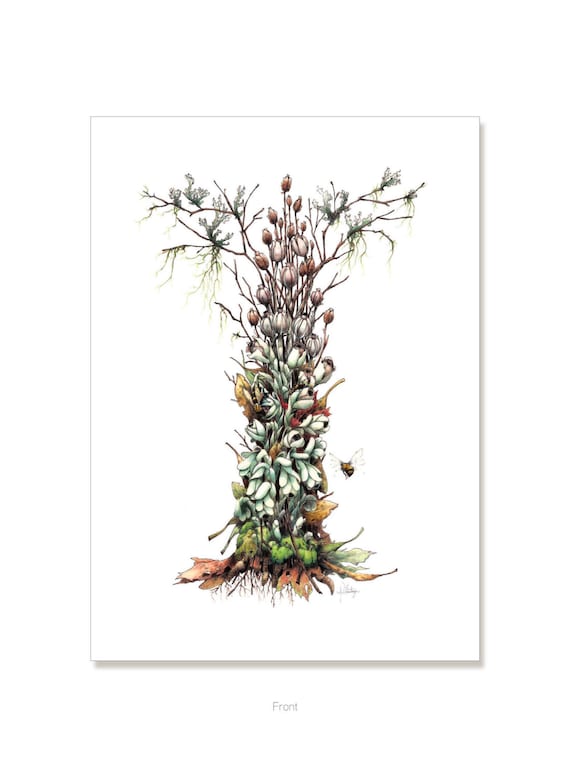This is an illustration of a plant positioned at the very bottom center of the image, labeled "front" in light gray. The artwork appears on what looks like a white piece of paper, with a very light gray outline and a slight shadow near the bottom and to the right, lending it a sense of depth. The plant itself is surreal and unlike any known species, featuring small roots at the base and a variety of flowers and buds extending upward. Its branches spread out horizontally to the left and right, with some resembling hanging roots or moss, adding to the alien-like appearance.

At the bottom right of the plant, a bee (or possibly a butterfly) hovers nearby but does not land. The lower portion of the plant displays green colors that transition to a lighter greenish-whitish hue towards the top, with the flower bulbs being white with a hint of pink. Brown stick-like branches jut out to the sides, adorned with green leaves. Additionally, the artist's signature can be found in the bottom right corner, although it is too small to decipher the name. The entire composition, set against the white background, gives a detailed and dimensional depiction of this otherworldly floral form.